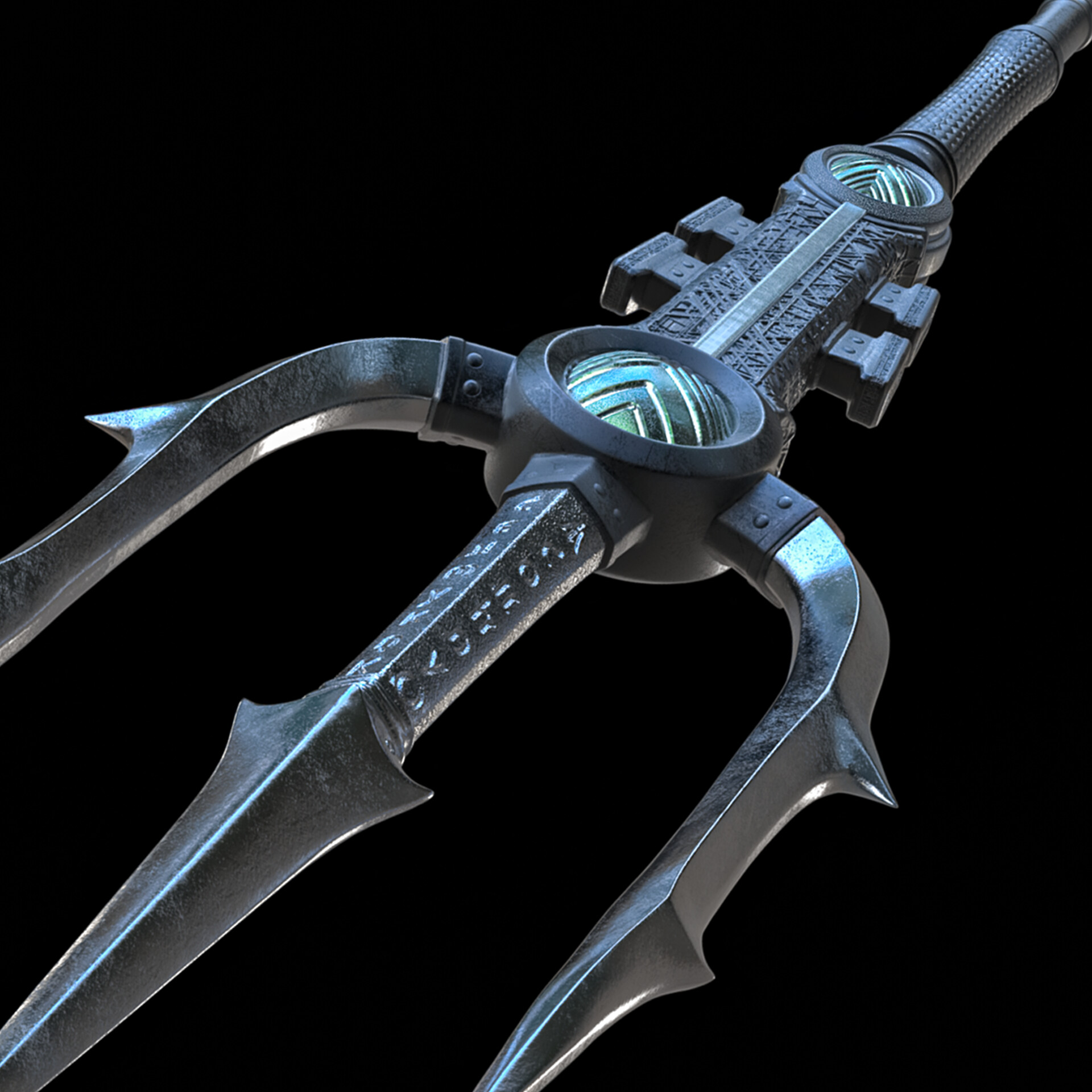The image depicts a highly detailed, futuristic trident set against a solid black background. The trident, possibly AI-generated and crafted from steel, showcases three prongs, each with jagged points. The central prong is notably sharp and double-edged. The handle features intricate carvings, including two circles etched with V-shaped designs highlighted in green. Further down, the handle is black with a rubber grip and has two knobs protruding. The weapon's elaborate design, including crisscrossing lines and engraved details on the metal, suggests it could be a prop from a fighting movie.